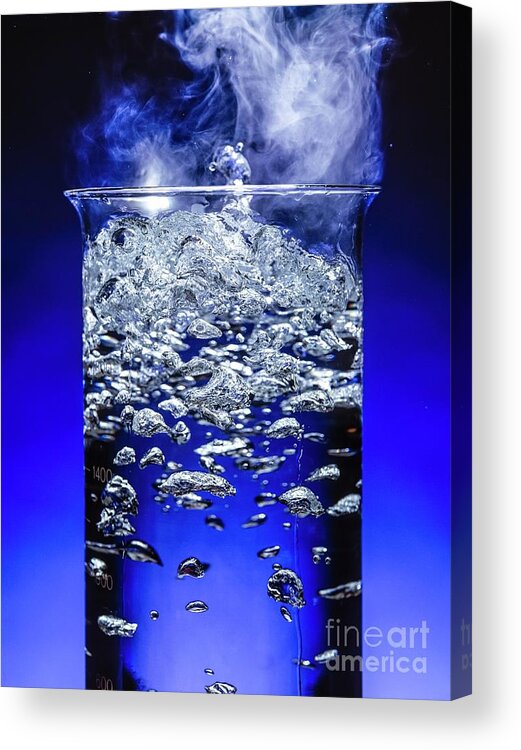The image features a striking piece of pop-up wall art displaying a 3D photograph that rises about two to three inches from the wall. At the center of the image is a close-up of a beaker containing a clear liquid, likely water, from which steam and heat bubbles emerge. The steam, initially white, takes on light lavender and blue hues as it ascends against the background. The water appears to be boiling, with vigorous coalescing bubbles at the top. The backdrop is a gradient that transitions from a dark blue at the apex to a lighter blue near the base, with hints of black near the top. In the bottom right corner of the photograph, the semi-transparent text "Fine Art America" is visible, suggesting a watermark.